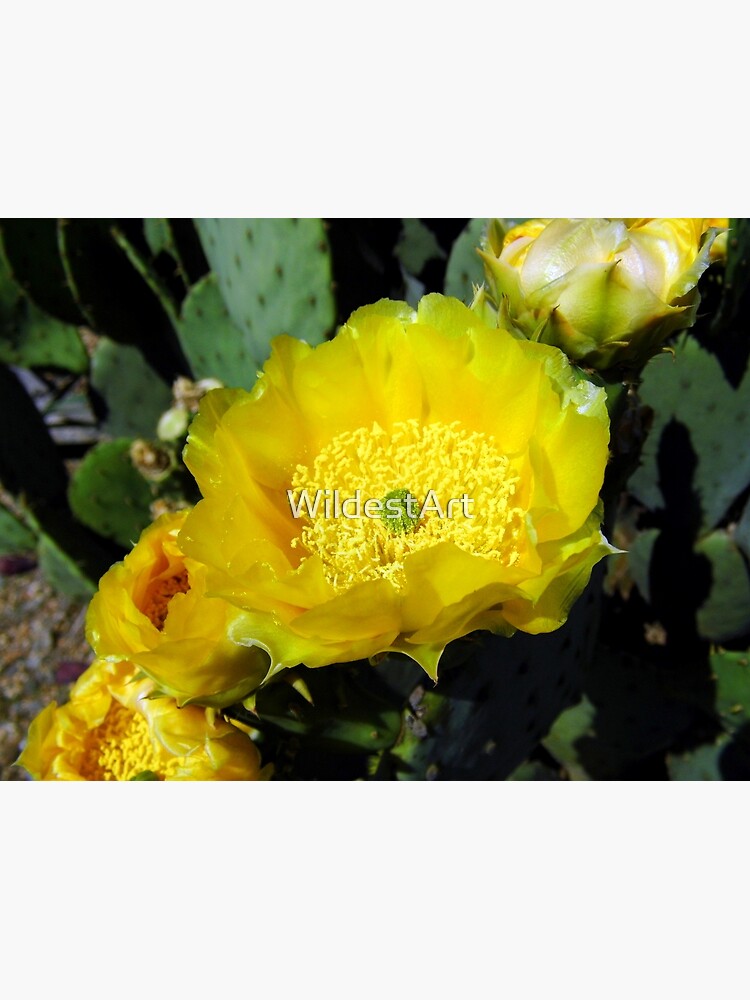This horizontal rectangular color photograph features a central large yellow flower with light greenish petals and a distinct round green spot in its middle. Superimposed on this flower is white text reading "Wireless Art." The background is deliberately blurred, revealing large oval cactus leaves with prominent spikes, casting shadows and adding to the textured backdrop. Yellow flowers are scattered throughout, with one positioned in the upper right corner and two more in the lower left corner, all contributing to the rich visual tapestry centered around the theme of natural beauty and artistic text.